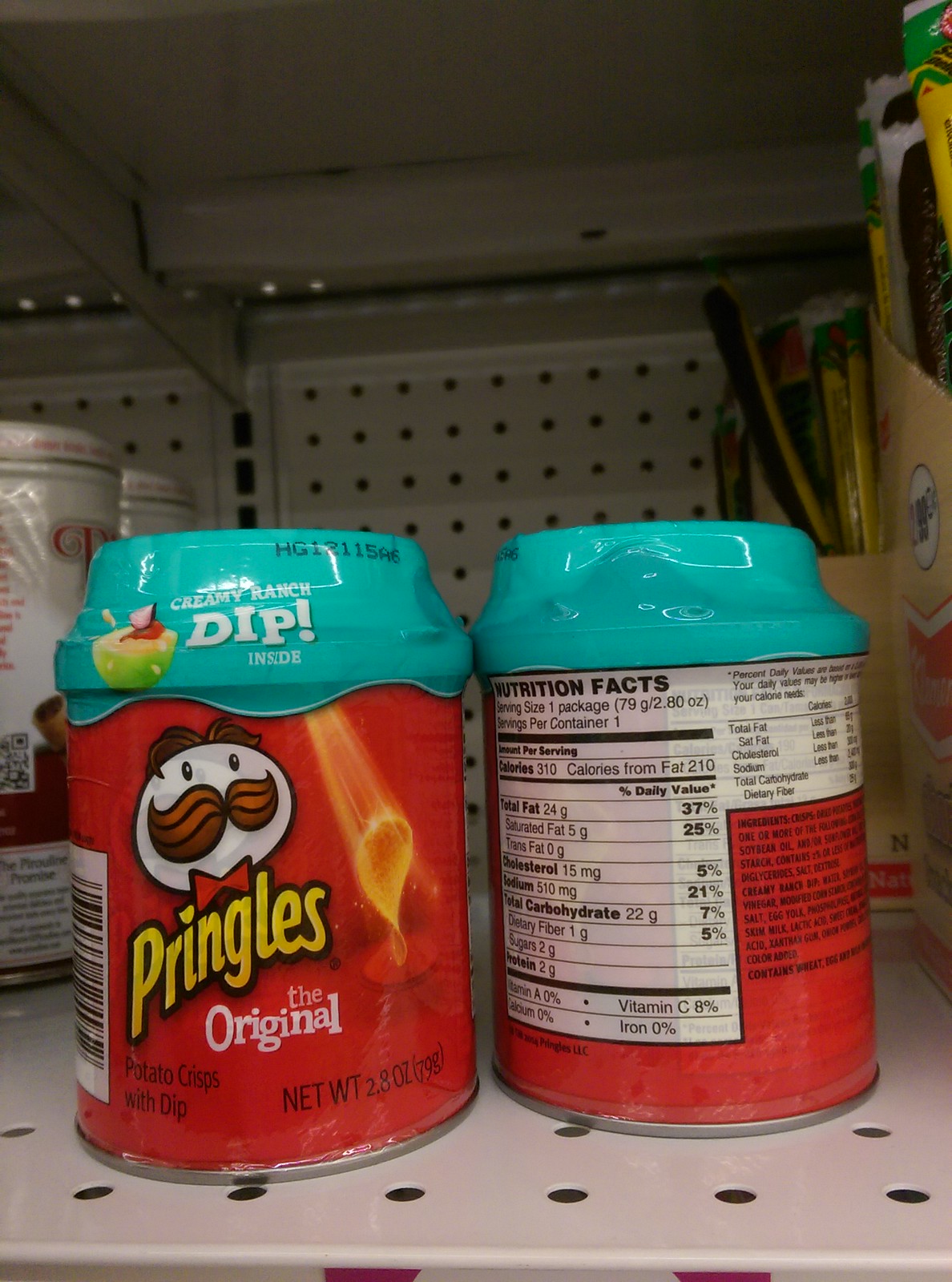On a metal shelf perforated with small holes, two notable canisters stand side by side. The first canister, prominently displayed on the left, is a vibrant red Pringles can branded with its iconic "Original" flavor. This canister is topped with a contrasting turquoise lid, which is adorned with an additional label promoting a "Creamy Ranch Dip"—suggesting an integrated dip add-on to complement the Pringles. To the right of it, an identical Pringles canister is positioned with its back facing forward, revealing its nutrition facts. Although the picture quality diminishes the legibility of the small-font nutrition details, the label is clearly visible. In the background, other canisters unfocus into obscurity, their labels and contents indiscernible.